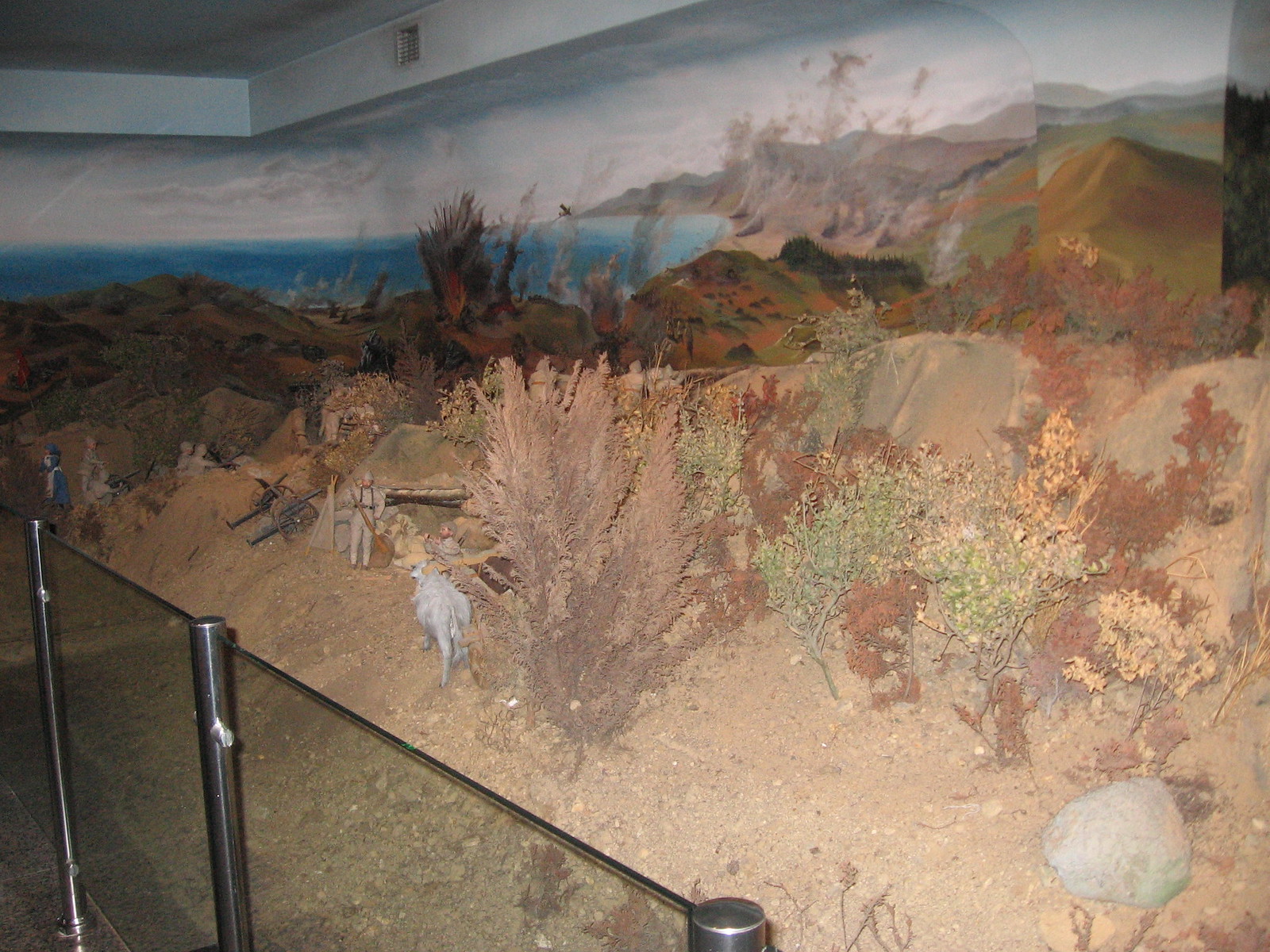The image depicts a museum exhibit designed to resemble a desert landscape with wild animals. The scene features sandy terrain with hills and rocky outcrops, interspersed with plants that are brown, yellow, and green in color. The exhibit includes a life-sized diorama setup with realistic elements such as bushes and rocks. In the background, a mural extends from the top half of a wide, rectangular-shaped wall downwards, curving around to the adjacent wall. This mural is intricately painted to blend seamlessly with the physical exhibit, showing an ocean and sky in the distance, rocky hills with rusty green grass, and additional sandy areas with brownish weeds. 

To protect the display, a glass railing is situated around it, along with dark grey metal poles that support a rope barrier. The actual wall beneath the mural appears to be a medium grey, marbled concrete. Notably, the exhibit also includes human figures, possibly in military uniforms, along with some carts, suggesting a historical or wartime context. The detailed, immersive setup and the protective glass block highlight the exhibit's importance and add to its lifelike appearance.